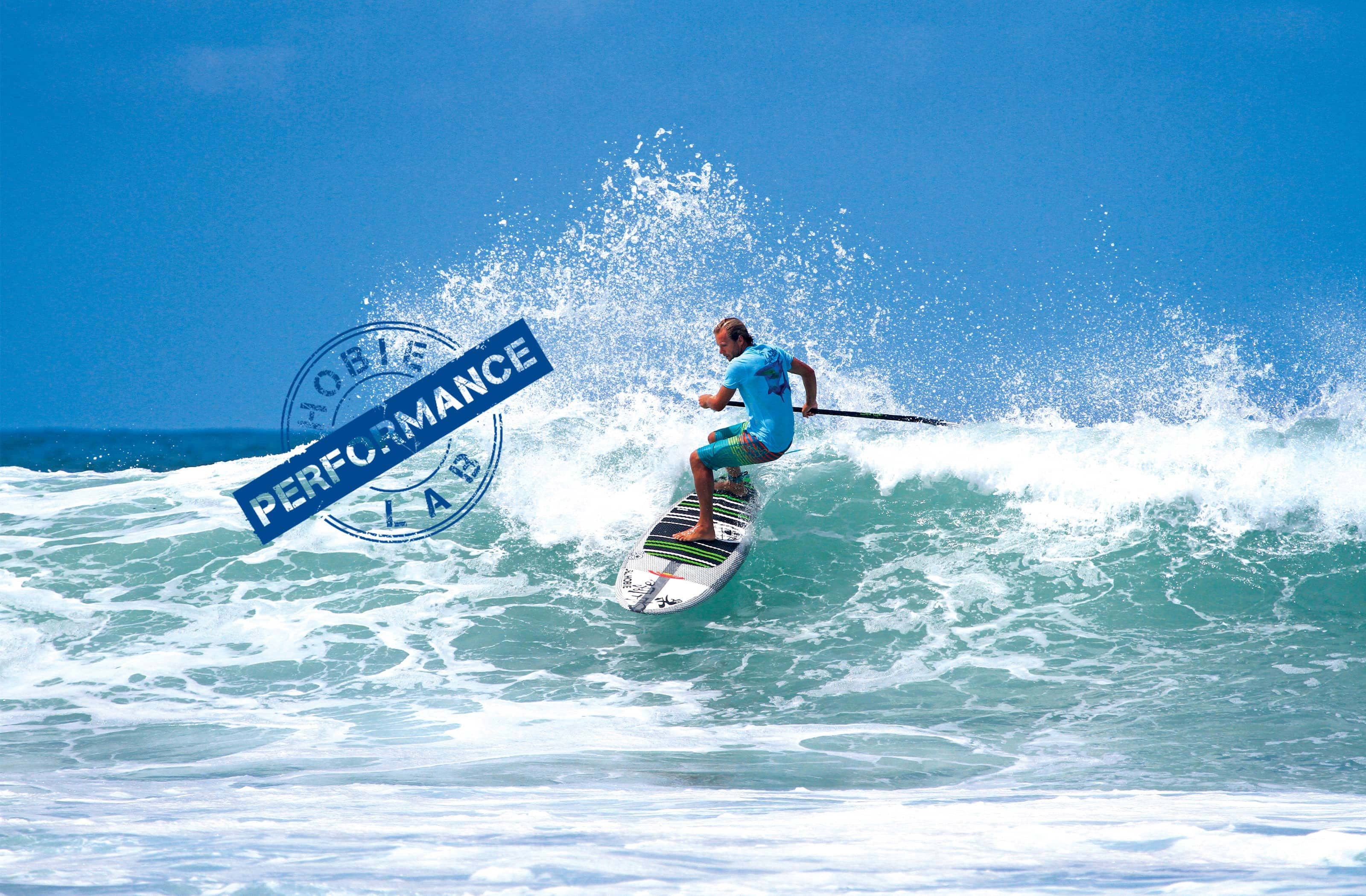In this wide-angle photograph, a surfer is captured riding a wave, balanced precariously at the top. The surfer, clad in a light blue short-sleeved t-shirt and vibrant multi-colored shorts transitioning through teal, green, yellow, and red, is holding a pole, likely a paddle, to maneuver through the waves. His surfboard is primarily white with green and blue stripes, featuring a textured patch for better foot grip. The ocean beneath him appears turquoise, lively with crashing waves that rise high, indicating strong movement and splash. The sky overhead is a deep, cloudless blue, adding to the serene yet dynamic atmosphere of the scene. To the left of the surfer, there's a watermark—a blue circle with a dark blue diagonal banner. It reads "Hobie" at the top of the circle, "Performance" across the banner, and "Lab" at the bottom, suggesting that the image could be part of an advertisement for Hobie Performance Lab. The surfer, soaking wet, appears to have already fought hard with the waves, embodying the vigorous spirit of surfing.